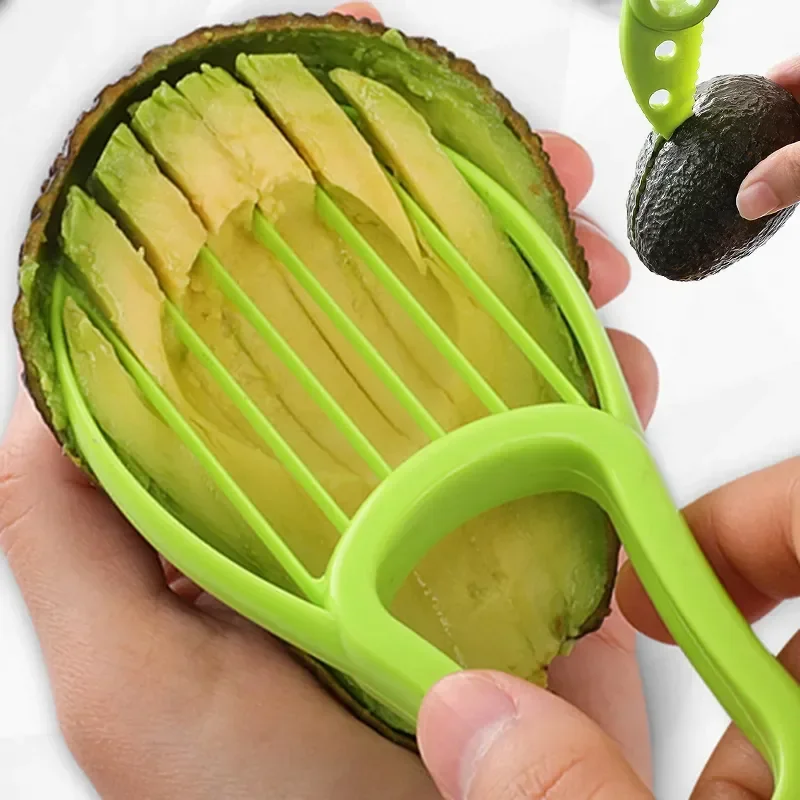In the image, a person is using a lime green, plastic grater-knife to scoop out the flesh from a halved avocado. The grater-knife, which has serrated edges and two holes in its blade, is adeptly peeling the inside contents of the avocado, which displays characteristic green and yellow hues. In the upper right corner, a smaller inset shows the person cutting another whole avocado in half with the same versatile tool. The close-up detail of the main image emphasizes the effectiveness of this multifunctional device, showcasing its ability to grate and slice the avocado into neat strips. The image conveys the tool's utility, perhaps suggesting its appeal in an infomercial context.